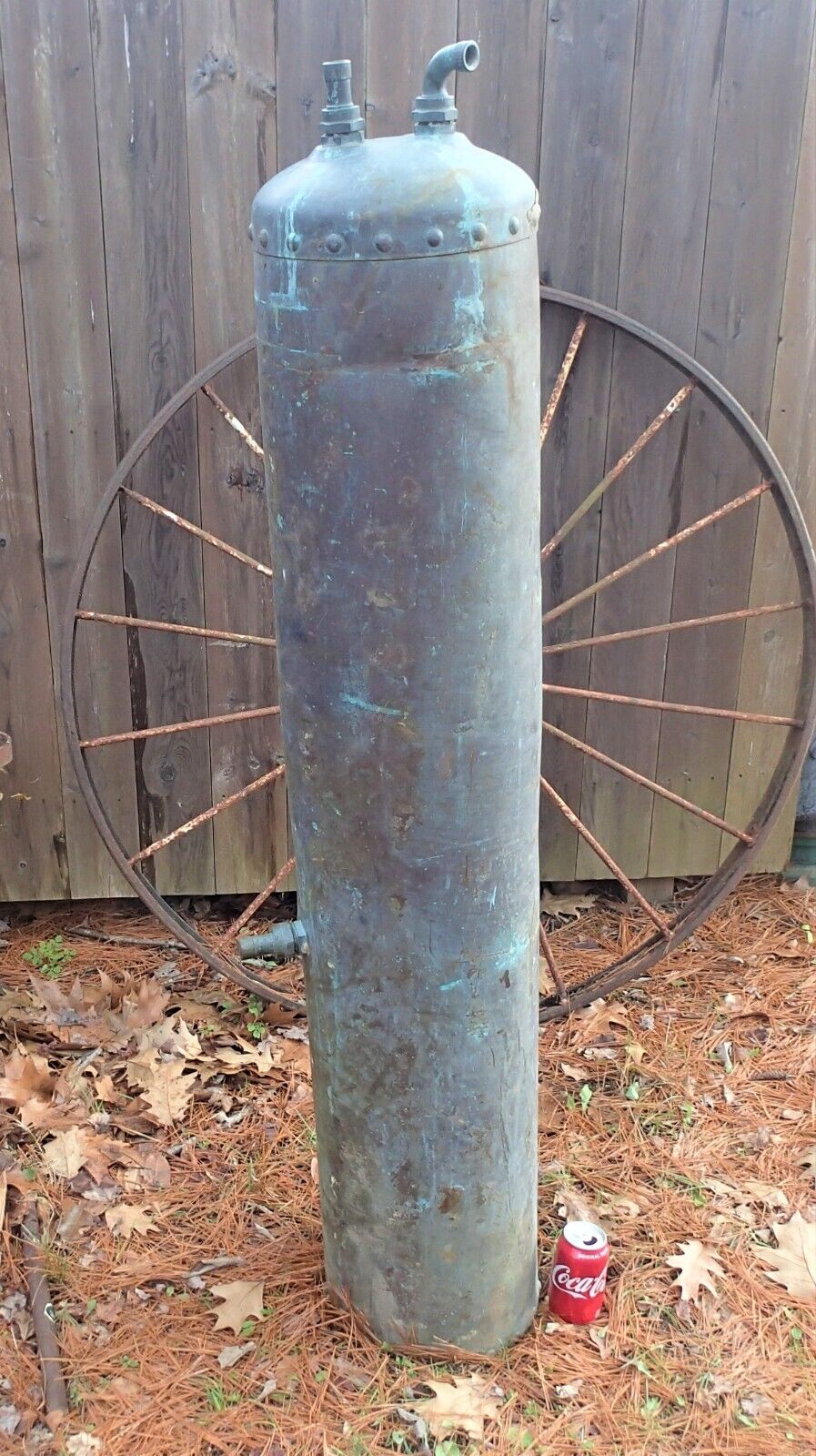In the daylight, a photograph captures a large, cylindrical metal canister, resembling an oversized oxygen or helium tank, standing prominently on a ground scattered with straw and leaves. The canister measures approximately five feet tall with a silver body marred by blue marks, numerous scratches, and a green patina, hinting at weathering and possible moss growth. Topped with a riveted cap, the canister features two spigot-like pipes: one extending straight up and the other curving at a 90-degree angle. Beside it on the ground, a red and white Coca-Cola can lies, helping to scale the canister's imposing size. Behind the canister, partially obscured, leans a large, rustic brown wagon wheel against a wooden wall, framing the scene in what appears to be a mountainous or rustic yard setting.